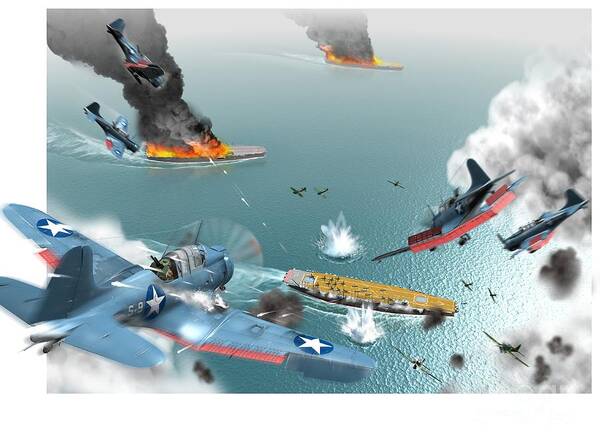In the image, we observe an aerial view of a dramatic battle scene rendered in digital art. Dominating the scene are several blue fighter planes, each adorned with white stars inscribed within blue circles on their wings and body. The tips of their wings at the rear are vividly painted red. These warplanes engage in intense combat, firing down onto a brown-colored ship amidst the blue, tranquil waters which have a slight teal hue. The impact of the shots creates large white splashes on the surface.

In the background, two ships are engulfed in dark black and lighter gray smoke, contributing to the dangerous and tense atmosphere. This smoke rises ominously into the sky, mingling with the light gray fog that covers the distant parts of the scene. On the left side of the image, one plane is positioned closest to the viewer and extends beyond the edge of the image, enhancing the visual depth with a 3D effect. The serene water contrasts sharply with the chaos of the battleground, making the action more pronounced against the otherwise still surface. Overall, the digital rendering powerfully captures the intensity and peril of this aerial and naval clash.